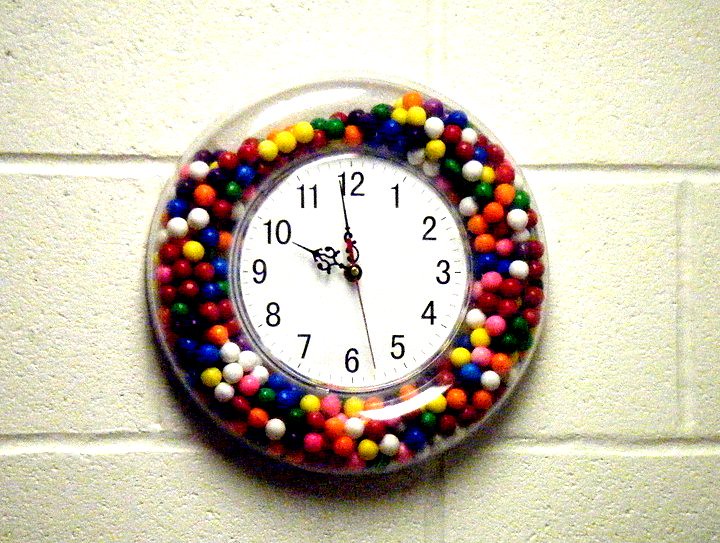This color photograph captures a unique ornamental novelty wall clock mounted on a greyish-yellow brick wall, likely influenced by artificial lighting affecting its hue. The clock features a round face with a white background and black numerals. Surrounding the clock is a transparent, circular container, made of either plastic or glass, filled with numerous small, spherical balls. This container encircles almost the entire clock face except for a segment at the upper left portion, which appears empty and void of the balls.

The clock's hands are distinctly visible: the hour hand points to 10, the minute hand is nearing 12, and the second hand rests between 5 and 6. The intricate detailing of the minute hand includes an ornamental round design, adding to the clock's decorative appeal. The artificial lighting shining down on the clock enhances the visual curiosity of this novelty timepiece against the textured background.